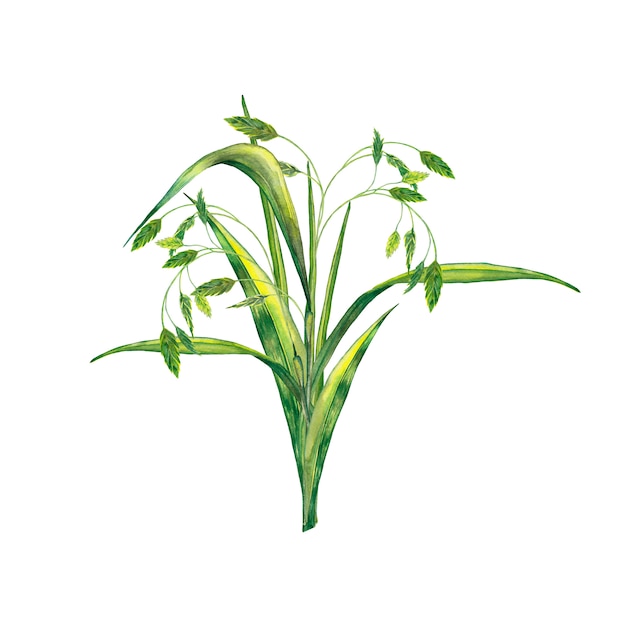This detailed, colored pencil illustration depicts a mature, green plant against a plain white background. The plant, possibly resembling oats or a similar species, is rendered with varying hues of green, ranging from dark to light. It features a central stem that becomes pointy at the base and tapers out with larger, pointy leaves extending to the sides. Additionally, there are 8 or 9 feathery, smaller stems bending outward, heavy with the weight of their small, leaf-like structures at the tips. The drawing captures a realistic shading effect, enhancing the depth and natural appearance of the plant. There are no flowers, text, or background details present in the image.